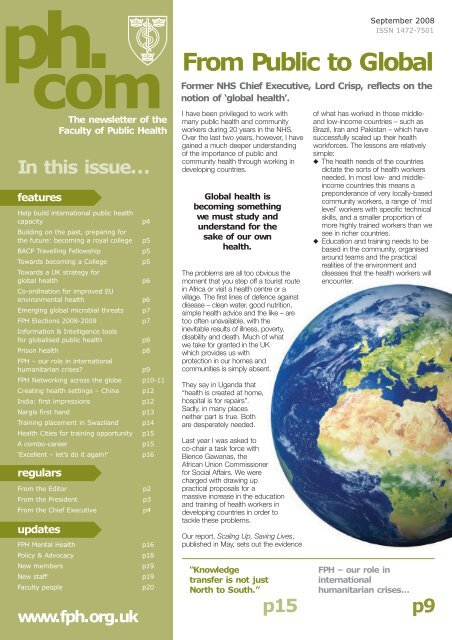This image appears to be an advertisement or cover for a publication. At the top-left corner, there's a lowercase web address: "ph.com" with a medical symbol featuring a snake entwined around a pole on a shield. Below this emblem, in white print, it reads, "The Newsletter of the Faculty of Public Health." In beige print, there's a heading that says "In This Issue..." followed by a list of featured articles, each accompanied by a page number, which extends down the page. There is also a section labeled "Regulars and Updates." The website "www.fph.org.uk" is prominently displayed.

On the right-hand corner of the image, it indicates the publication date as "September 2008," with an associated ISSN number right below. In greenish print, a heading states, "From Public to Global," with an accompanying article filled with several paragraphs of text. Towards the bottom-right corner of the image, there's a detailed picture of the Earth, showcasing vibrant views of water, land, and clouds.